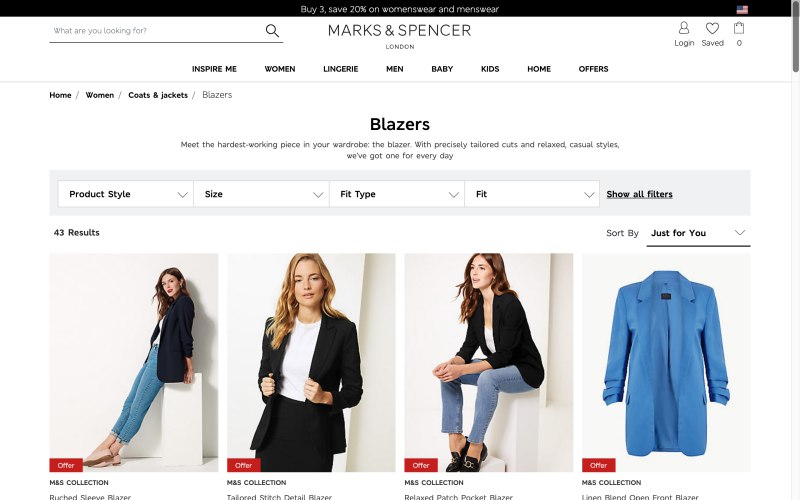This image depicts a webpage from the Marks & Spencer website, known for its women's and men's wear. At the very top of the page, there is a long, skinny black rectangle with white text that reads, "Buy 3, Save 20% on Women's Wear and Men's Wear." Directly below this banner is a search bar labeled "What are you looking for?" with a clickable search icon in the shape of a magnifying glass. To the right of the search bar, there are options to log in, view saved items, and check the shopping bag, which currently displays "0" indicating no items have been added.

As you scroll down the page, there are clickable links for various categories including "Inspire Me," "Women," "Lingerie," "Men," "Baby," "Kids," "Home," and "Offers." Further down, specific sections for "Home," "Women," "Coats and Jackets," and "Blazers" are visible. The 'Blazers' section is currently selected, showcasing four blazers. Three images feature models wearing different blazers, while the fourth image presents a blazer on a hanger. All the items are from the "M&S Collection." The models elegantly display the blazers, giving potential buyers an idea of how they look when worn.